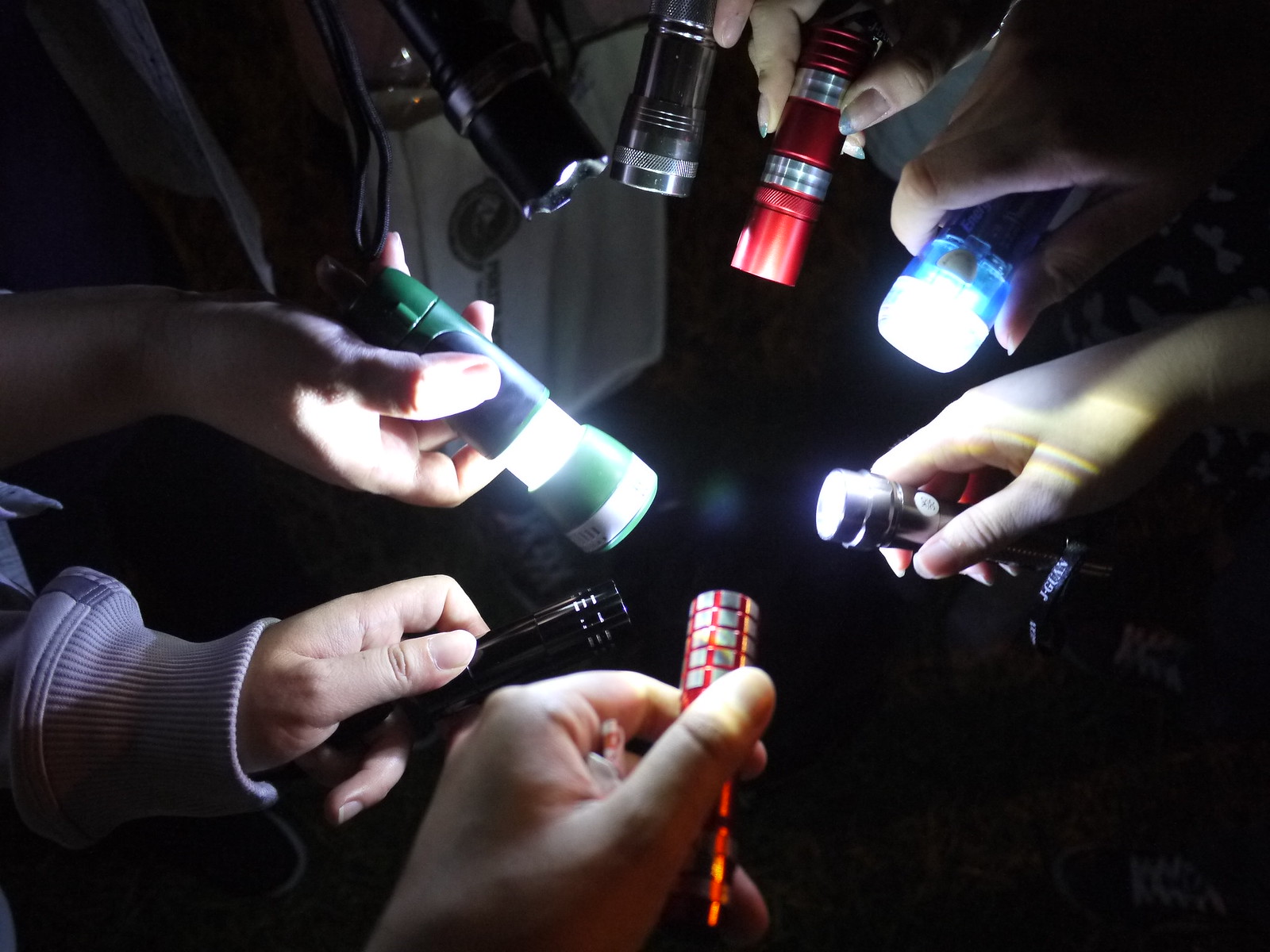This nighttime close-up photograph captures several hands, primarily of younger Caucasian individuals, forming a circle and holding various small, handheld flashlights pointed inward. The image is illuminated solely by the beams from these flashlights, creating a striking visual effect in the dark. The hands, mostly shown from the wrist down, feature different colored sleeves, including a noticeable purple cuff on the lower left. The flashlights vary in color and style; notable ones include a red flashlight in the bottom center, another red one at the top center, a blue flashlight on the upper right, and a green one on the left. Additionally, silver and black flashlights are scattered throughout the circle, with the brightest beams shining from the lights at approximately 3 o'clock and 9 o'clock positions. The unique arrangement of hands and lights creates a captivating, illuminated circle against the darkness.